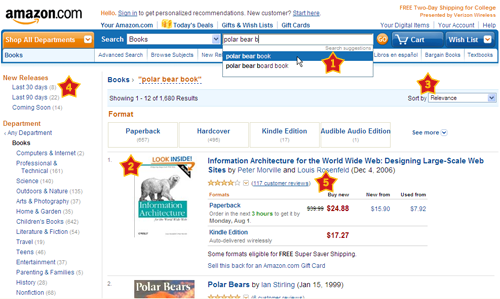The image displays an Amazon.com webpage prominently featuring various elements and features available to users. At the top of the page, there is a gold arrow accompanying a message that reads, "Hello, sign up to get personalized recommendations. New customer? Start here." Adjacent to this, there are navigation options labeled "Today's Deals," "Gift and Wish Lists," "Gift Cards," "Your Digital Items," "Your Account," and "Help." 

Highlighted in gold at the top, a banner promotes "Free Two-Day Shipping for College" presented by Verizon Wireless. 

Beneath this, a tab spans across with two layers of categories. The leftmost category reads "Shop All Departments," and underneath, there is a dropdown for "Books" with options for an advanced search, browsing subjects, and performing a book search.

Currently, the search is set to "books," and the keyword "polar bear book" has been entered, returning a recommended result for a "Polar Bear Board Book." The search results are marked by a large star, indicating a notable recommendation. 

The cart icon shows no items, and there are suggestions for new releases and additional book department categories listed on the side.

Among the search results, the image mentions that it is one of 12 listings on the first page. Notably, the first book listed, titled "Information Architecture for the World Wide Web: Designing Large-Scale Web Sites," seems unrelated to polar bears, causing some confusion. The second book in the results, however, is relevant to polar bears. The incongruity of the first listing is humorously noted.